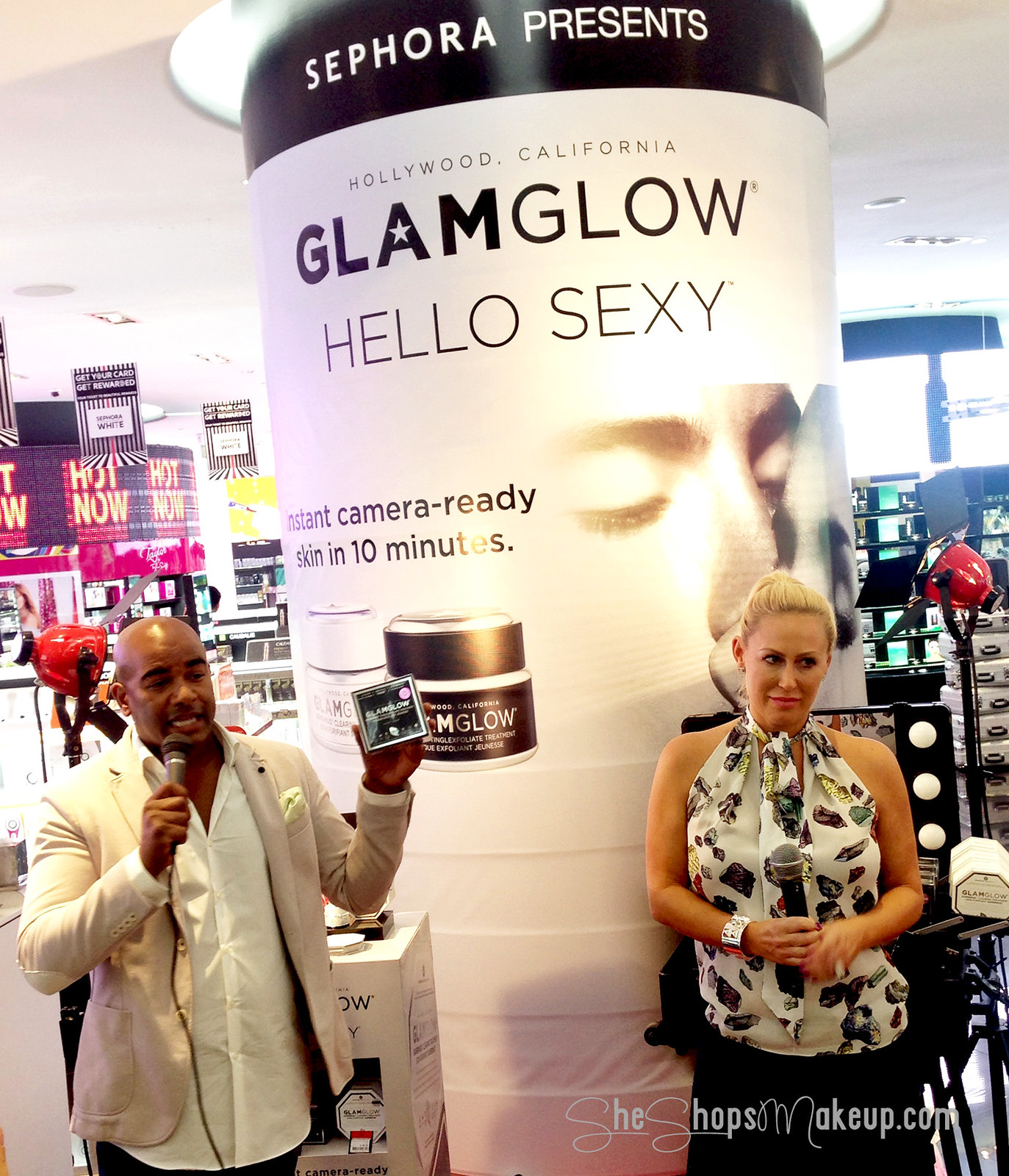At what appears to be a makeup convention or store event, a bald African American man with a goatee, dressed in a white untucked button-up shirt under a beige blazer, and a blonde Caucasian woman with her hair tied back in a bun, wearing a patterned short-sleeve blouse that exposes her shoulders, stand side by side, each holding a microphone. The man, clutching a square object in his left hand, and the woman, with a large bracelet on her right arm, pose in front of a towering cylindrical display. The cylinder reaches the ceiling, touching a lit circle, and bears the words "Sephora Presents" in a black band at the top. Below this, on the white section, are the phrases "Hollywood, California, Glam Glow, Hello Sexy," followed by "Instant camera-ready skin in 10 minutes" near an image of a brown jar labeled "Glam Glow." The scene is detailed with background signs and displays, with a decorative website inscription, SheShopsMakeup.com, visible in the bottom right corner.